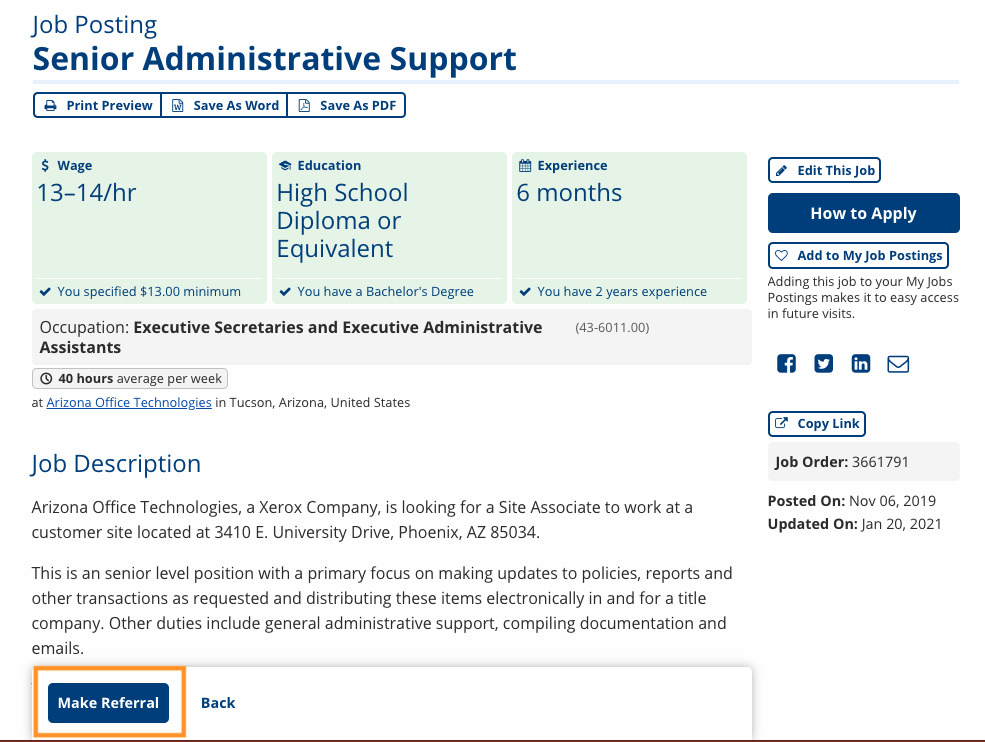**Job Posting Screenshot: Senior Administrative Support**

This screenshot details a job posting for a **Senior Administrative Support** role, highlighted in bold blue letters. There are options to view a print preview, save the posting as a Word document, or save it as a PDF.

Highlighted in three mint green rectangular areas side-by-side are the following details:
- **Wage**: $13 to $14 per hour (Minimum wage specified: $13)
- **Education**: High school diploma or equivalent required (Bachelor's degree noted)
- **Experience**: Minimum of 6 months required (2 years experience noted)

**Occupation**: Executive Secretaries and Executive Administrative Assistants  
**Hours**: 40 hours per week  

**Company**: Arizona Office Technologies (a Xerox company)  
**Location**: 3410 East University Drive, Phoenix, Arizona, 85034  

**Job Description**:  
The Senior Administrative Support position at Arizona Office Technologies focuses on updating policies, reports, and other transactions as requested. These must then be distributed electronically to a title company. Other duties include general administrative tasks, report compilation, documentation compliance, and managing emails.

At the bottom of the job posting is a yellow-highlighted button for referring someone to the job. In the upper right corner, there is an "Edit This Job" button. Below that are buttons marked "How to Apply" (in blue) and "Add to My Job Postings." There are also social media icons for sharing on Facebook, Twitter, LinkedIn, and emailing the job posting. Additionally, there is an option to copy the job link and a button to show the job posting's order, along with information about when it was posted and last updated.